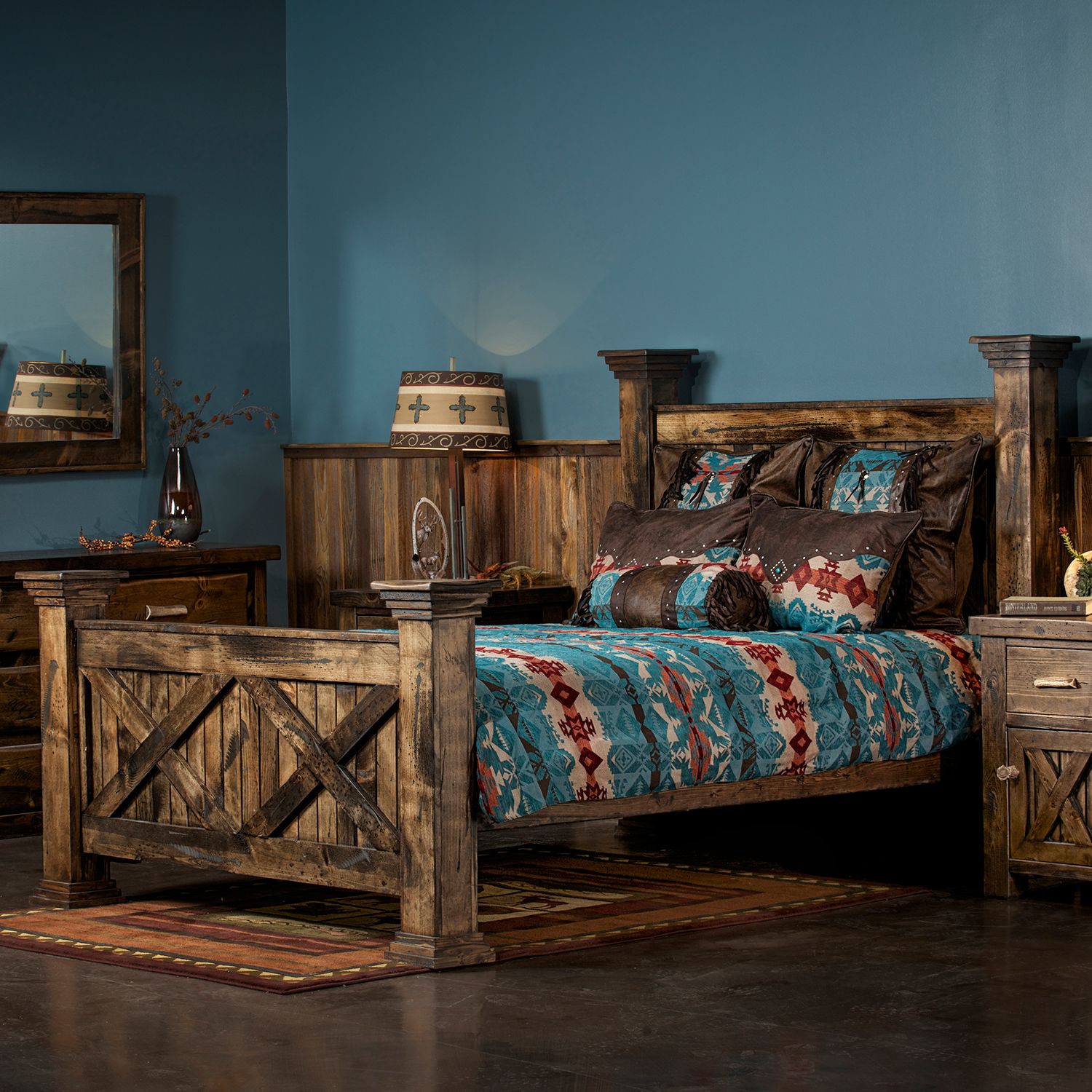The image depicts a neatly organized bedroom with blue painted walls, featuring a large, angled wooden bed adorned with a southwestern-style quilt in colors of blue, red, orange, and tan, accompanied by matching pillows and shams. The bed's headboard and footboard have a distinctive design with rectangular posts and “X” patterns. On each side of the bed, there are matching wooden nightstands that complement the bed’s wood finish. Positioned on the left wall is a framed mirror, while a wooden dresser sits to the left of the bed, topped with a brown vase filled with coordinating flowers. The floor features a brown, tile-like appearance with a burnt sienna and reddish rug underneath the bed, adding warmth to the room's overall ambiance. A lamp can be seen in the background on the left side, providing additional detail to the cozy, well-coordinated decor. The photo, square in shape, captures the essence of a stylish, magazine-worthy bedroom with a blend of blue, brown, and tan hues throughout.